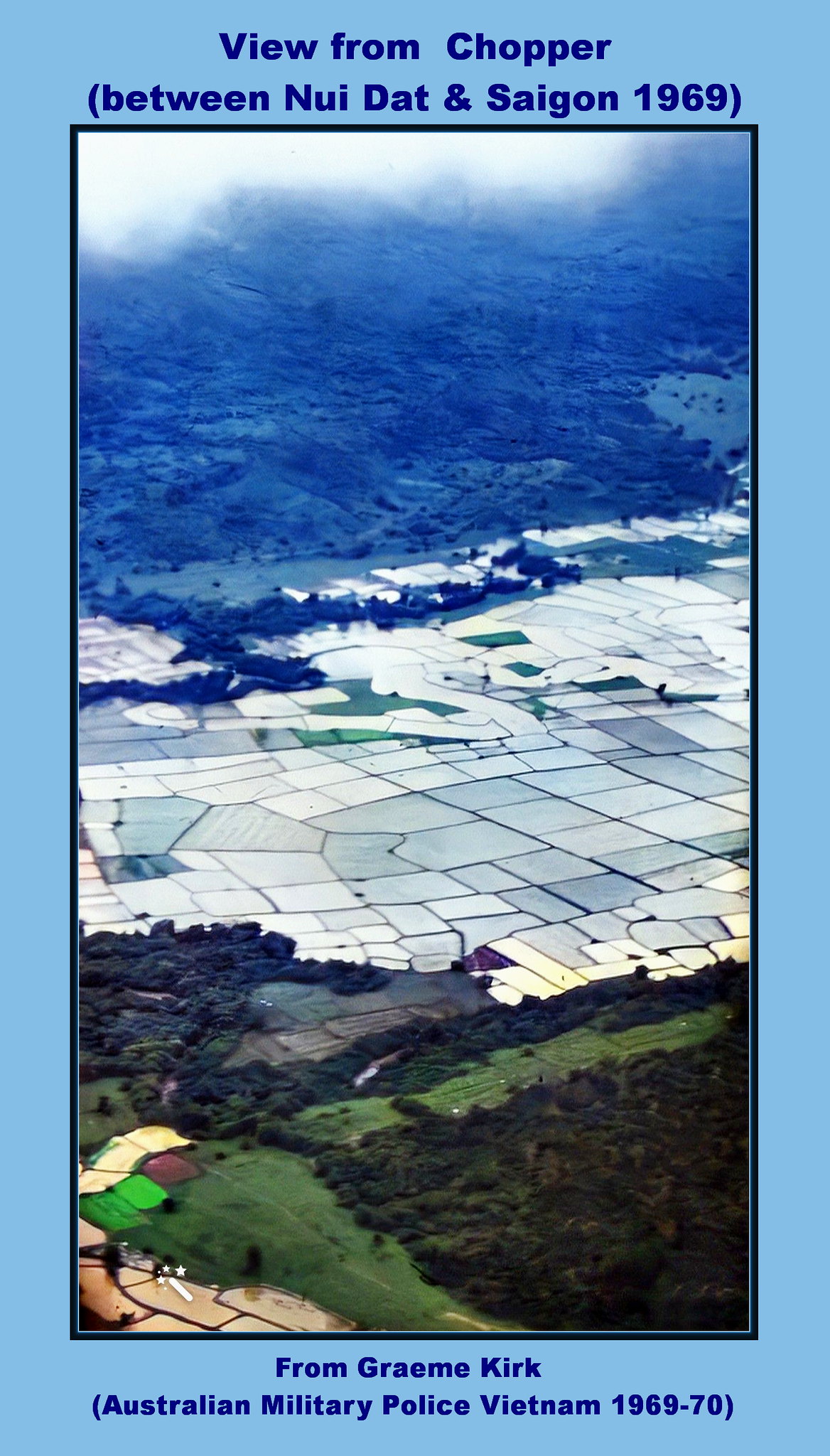The image is an aerial view, taken from a helicopter, showcasing the landscape between Nui Dat and Saigon in 1969. The scene captures an expanse of farmland divided into multiple square plots, interspersed with a variety of green spaces including dense patches of trees and shrubs. Prominent in the background is a rugged terrain that resembles a mountain or rocky outcrop. The image is framed with a light blue border, with dark blue text at the top reading "View from Chopper (between Nui Dat and Saigon, 1969)," and similar text at the bottom that states, "From Graham Kirk, Australian Military Police, Vietnam, 1969-70." The scene is set on a partly cloudy day, providing a clear view of the agricultural and natural features below.